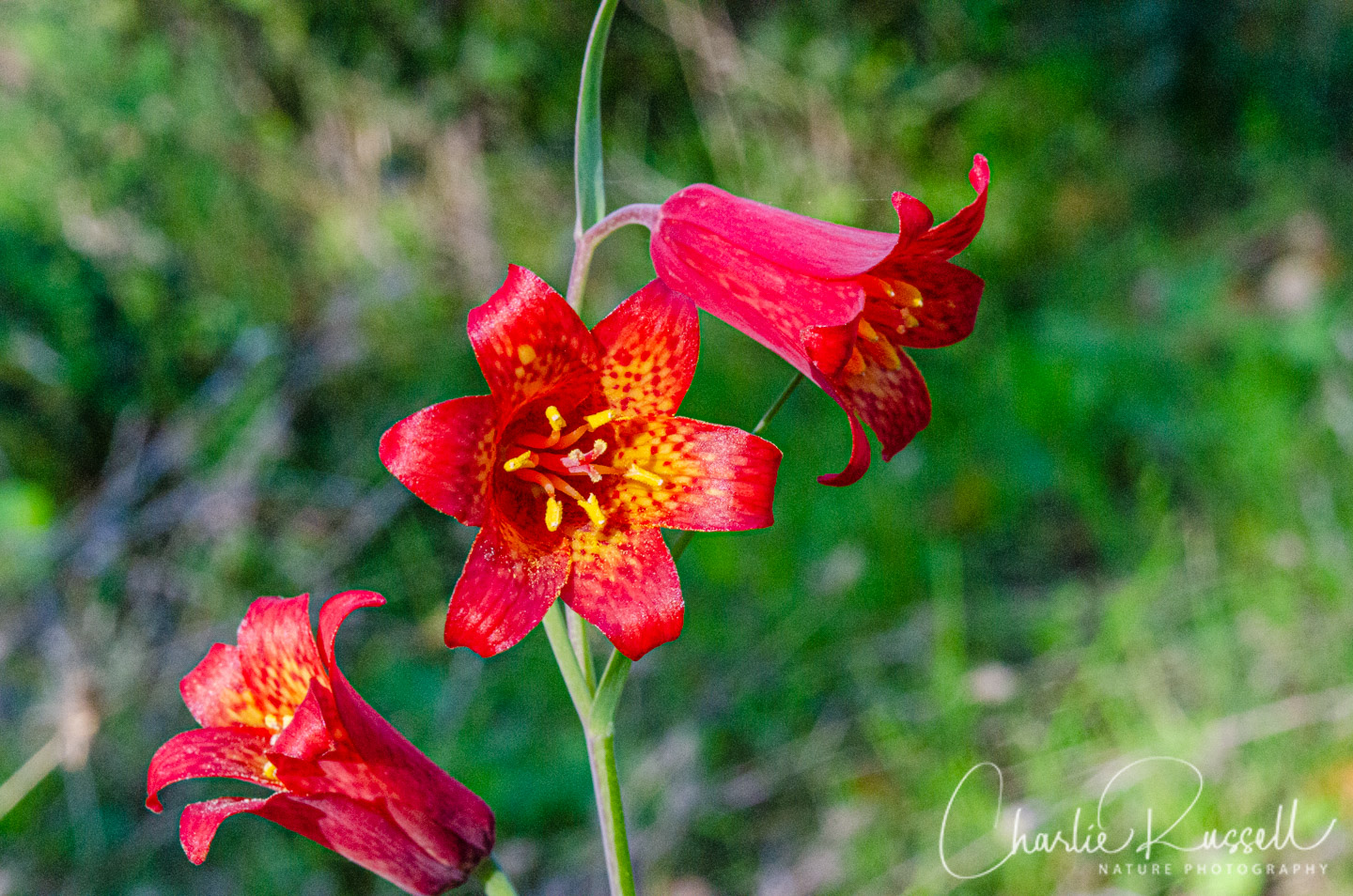This photograph by Charlie Russell Nature Photography captures the vivid beauty of three red-pink flowers, each adorned with six petals. They are artistically arranged on a single, thin green stem that stands vertically just off-center toward the left of the image. The focal flower, fully in bloom, faces forward at the center of the composition, revealing a striking gradient from its bright pinkish-red petals to a yellow-speckled interior. Flanking it are two slightly less open flowers: one positioned higher, angled downward to the right, and the other lower, facing the top right. Both of these flowers are still in their budding stages. Their yellow-tipped pistils add an extra layer of detail and contrast to the overall composition. The background is a soft blur of green, suggesting foliage and enabling the vibrant flowers to stand out prominently. At the bottom right of the image, the watermark "Charlie Russell Nature Photography" is elegantly inscribed, grounding the viewer in the artistry of the capture.